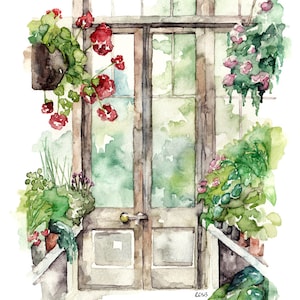This is a detailed watercolor illustration depicting the French doors of a greenhouse setting. The double doors, framed in brown, feature translucent glass panes with the hint of abstract greenery visible through them. Surrounding the doorway, the scene is adorned with various potted plants. 

In the upper left quadrant, a hanging plant with vibrant red flowers cascades down, its pot clearly visible. To the upper right, another hanging plant showcases lush greenery interspersed with delicate pink flowers that appear to spill out of their hidden pot. The lower right features more pink flowers amidst abundant greenery, all housed in classic clay pots. On the lower left, a collection of tall grasses and subtle purple blooms add to the verdant display.

Two railings lead up to the door, enhancing the greenhouse's inviting entrance. Above the doors and to the sides, additional panes of glass further integrate the interior with the surrounding natural beauty. The artwork beautifully captures the serenity and organic charm of this greenhouse scene.